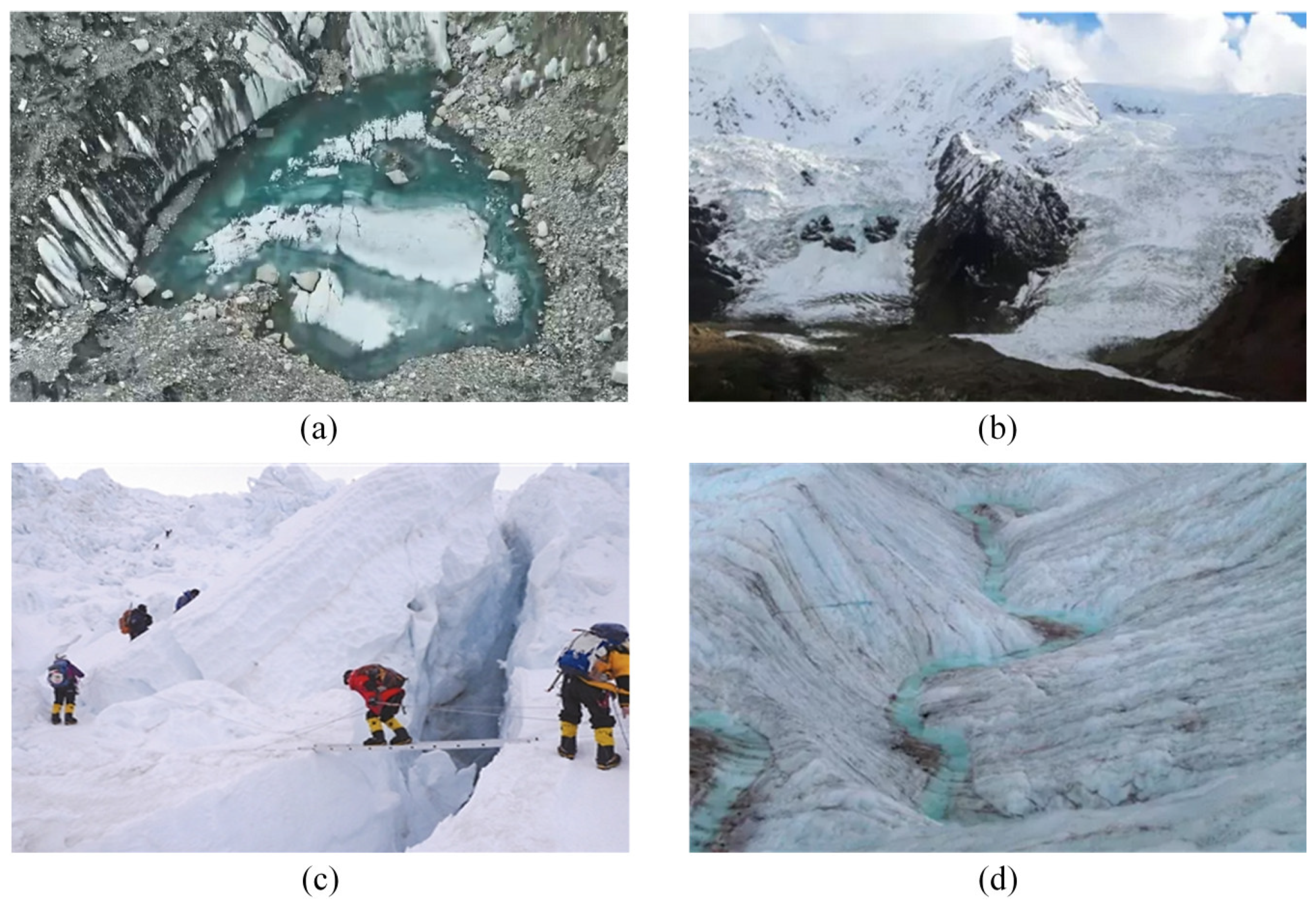The image consists of four separate photos labeled A, B, C, and D, arranged in a grid against a white background with two images at the top and two at the bottom. All depict various facets of a glacier landscape. 

- **Photo A (top left)** displays a glacial lake teeming with floating ice chunks, indicative of ice breaking apart. The clear aqua-blue water amidst the icebergs contrasts vividly against the white of the glacier.
- **Photo B (top right)** captures the snow-covered peak of a glacier, with patches of brown earth emerging as the snow melts. This aerial shot also reveals parts of the sky with scattered clouds.
- **Photo C (bottom left)** portrays climbers dressed in arctic gear navigating a snow-covered mountain. Two climbers are seen crossing a crevasse using a ladder to bridge the gap, emphasizing the challenging terrain.
- **Photo D (bottom right)** provides a close-up view of dirty ice or snow forming a deep crevice, through which water appears to be flowing.

The entire collection, likely taken during daytime under natural light, chronicles the majestic and rugged features of a glacier, combining overhead perspectives and detailed ground-level viewpoints.